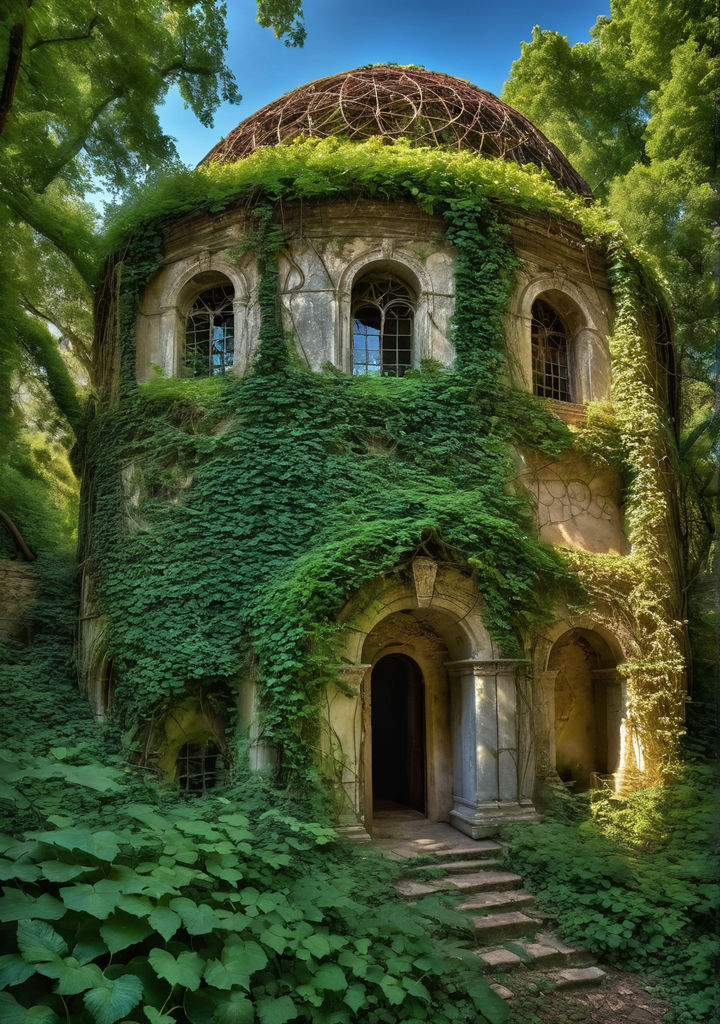The image depicts a large, cylindrical-shaped stone building with a distinct dome-shaped roof that appears almost nest-like or lattice-like in its intricate, intertwined pattern. The building is predominantly off-white or sandy in color, with weathered stone steps leading up to a black-brown front door flanked by two columns. Above the door, three arched windows are evenly spaced on the upper floor, while a single arched window is positioned on the ground floor. The entire structure is heavily adorned with ivy and lush green vines, suggesting nature's reclamation. Yellow ivy adds splashes of color against the lush greenery. The surrounding area is densely wooded, with tall green trees framing the scene, enhancing the secluded, forest-like setting. The sky above is stark white, suggesting the photo was taken during daylight hours under a bright, possibly overcast sky. The overall scene has an air of both abandonment and beauty, with nature overtaking the meticulously detailed stone structure.